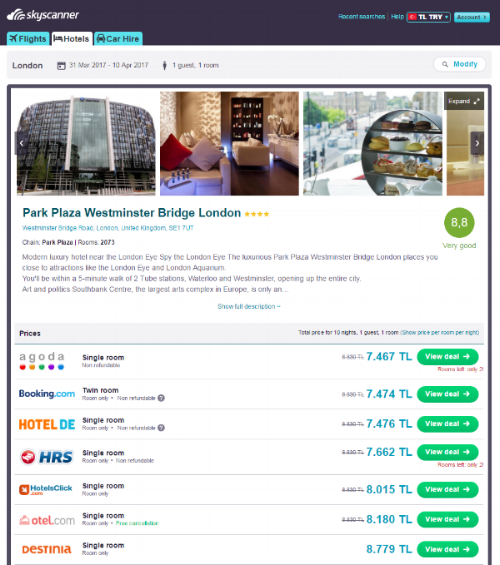In this image, presented at the forefront is a dark-themed interface labeled "Sky Scan" at the top left. The logo features white text accompanied by an image of a white cloud. Just beneath this title, three tabs are visible: "Flight," "Hotel," and "Car Hire." These tabs are primarily blue, except for the "Hotel" tab, which is white, indicating it is selected. 

Along the top right of the interface are additional tabs labeled "Recent Searches," "Help," "TL," "TAIL," and "Account." Below these, the destination "London" is prominently displayed, signifying searches for hotels in London. The search parameters are further detailed: dates from March 1, 2017, to April 10, 2017, for one guest in one room. A blue button labeled "Modify" is positioned to the right.

The main content of the page showcases the “Park Plaza Westminster Bridge London,” a 4-star hotel with yellow stars and the hotel name depicted in dark blue text. It is highly rated at 8.8 ("Very Good," written in green) and located at "Westminster Bridge Port, London, Tunisia, United Kingdom."

The hotel description highlights its modern luxury and proximity to iconic landmarks such as the London Eye and the London Aquarium. It emphasizes the convenience of being within a five-minute walk from Waterloo and Westminster Tube stations, making the entire city accessible. The description also mentions the South Bank Centre, Europe's largest arts complex, which is nearby. A green button labeled "Show Full Description" offers additional information.

Below this description, various booking options with associated prices are listed from different booking platforms: 

- Agoda: 7,467 TL
- Booking.com (Twin Room): 7,467 TL
- Hotel.de (Single Room): 7,467 TL
- HRS (Single Room): 7,662 TL
- Hotelclick (Single Room): 8,015 TL
- Hotels.com (Single Room): 8,180 TL
- Destinia (Single Room): 8,779 TL

Each option features a blue pricing detail and a green button labeled "View Deal" on the right side, allowing users to explore booking options.

This detailed caption provides a comprehensive overview of the interface, hotel features, and available booking options.